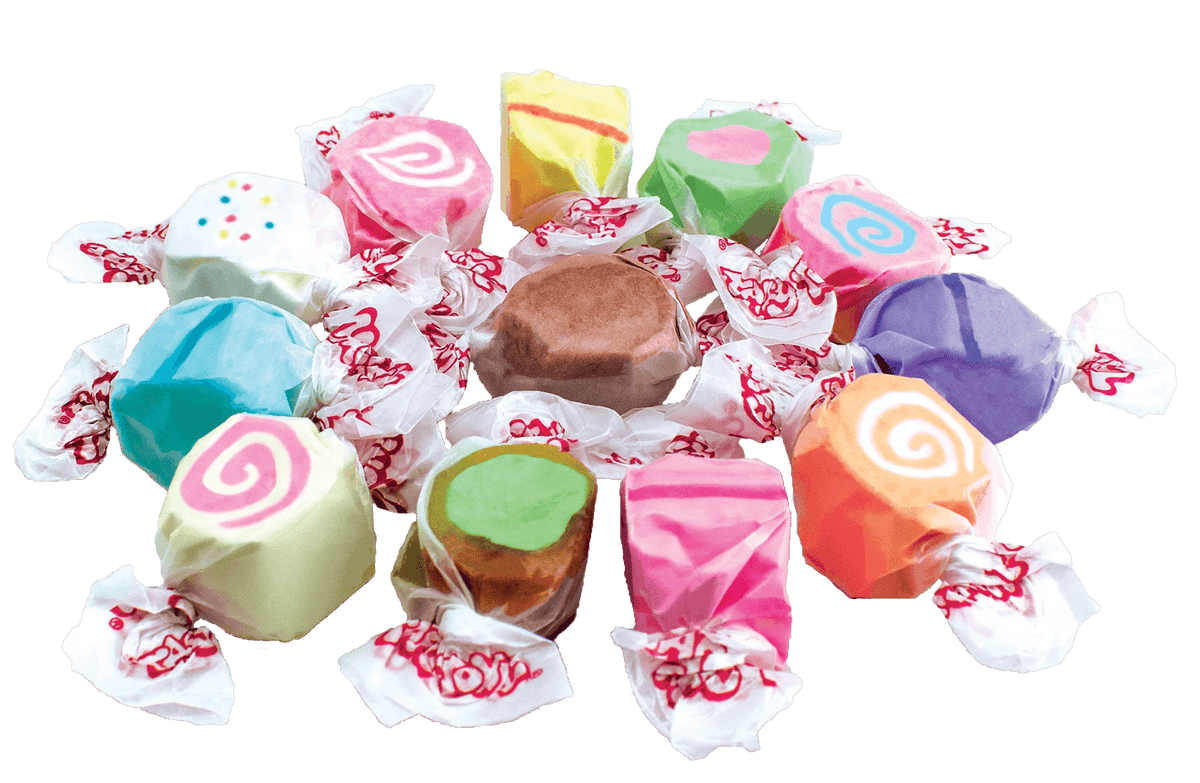The image features an assortment of colorful taffy candies, each intricately wrapped in white parchment-like paper adorned with red squiggly lines on each side. The candy arrangement is centered around a brown piece of taffy, forming a circular pattern outward. The variety of taffies includes:

- A white taffy with a pink swirl situated at the bottom left.
- A brown taffy with a green center.
- A pink taffy.
- An orange taffy with a white swirl.
- A completely purple taffy.
- A pink taffy with a blue swirl.
- A green taffy with a pink center.
- A yellow taffy with a red stripe.
- Another pink taffy with a white swirl.
- A white taffy with confetti-like polka dots.
- And finally a blue taffy.

The background of the image is white, enhancing the vibrant colors and designs of the taffies.